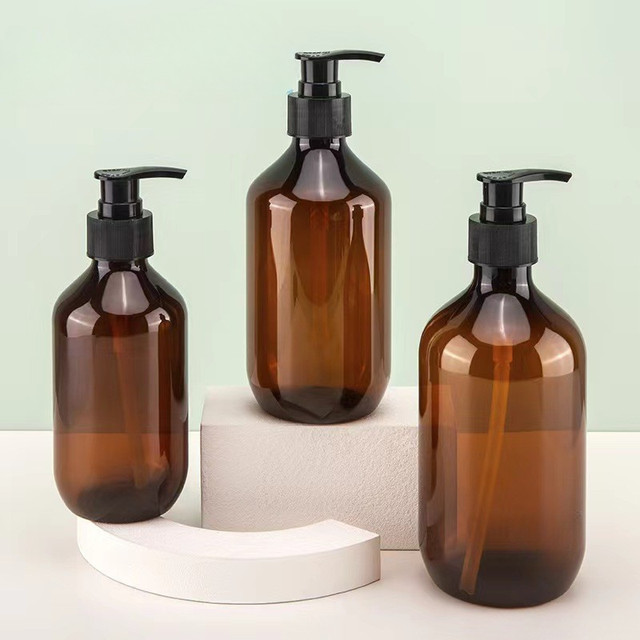The image features a detailed product setup of three amber-colored, semi-transparent bottles arranged on a white tabletop, with a light mint green background. All three bottles are of different sizes but share the same cylindrical shape. They are equipped with black, twist-on pump dispensers at the top, through which the contents—potentially lotion, shampoo, oil, or hand sanitizer—can be dispensed. These bottles are also see-through, revealing the internal tubes that reach down to the base for fluid suction. 

The smallest bottle is positioned on the left side atop a smooth, curved white stand, with its rounded bottom and flat sides leading up to the pump. The middle-sized bottle sits on a rectangular white stand with a concrete texture, slightly larger than the one on the left but identical in shape. The largest bottle, or the one potentially closer to the camera to appear larger, rests directly on the white tabletop. The arrangement and the clean, minimalist aesthetic of the setting highlight the bottles' functional yet elegant design.